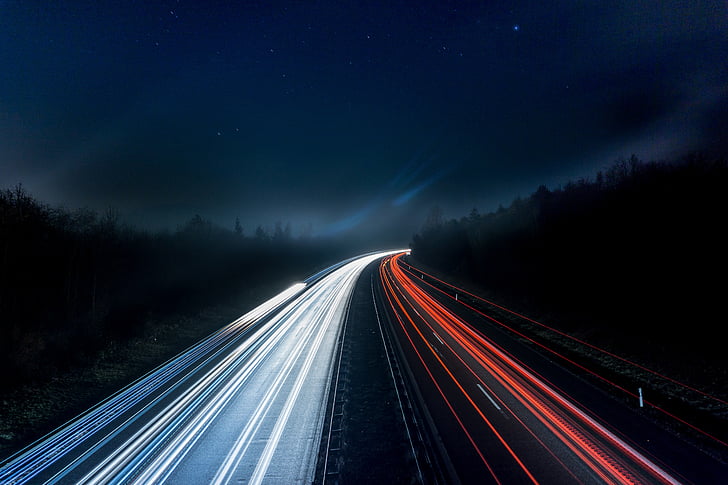This is a time-exposed photograph of a two-lane highway at night, possibly located in a wilderness area or mountains. The sky is a deep dark blue adorned with stars and streaky clouds that resemble the aurora borealis, giving the background an ethereal quality. On either side of the road, the darkness obscures hills and vegetation, allowing only faint outlines to be seen. The highway features white streaks of headlights on the left side, indicating vehicles coming towards the camera, and red streaks of taillights on the right side, showing vehicles speeding away. The light trails from the headlights and taillights dominate the scene, emphasizing the sense of fast movement through the night. The absence of visible vehicles is a hallmark of the long exposure technique used in capturing this image, enhancing its captivating and surreal nature.